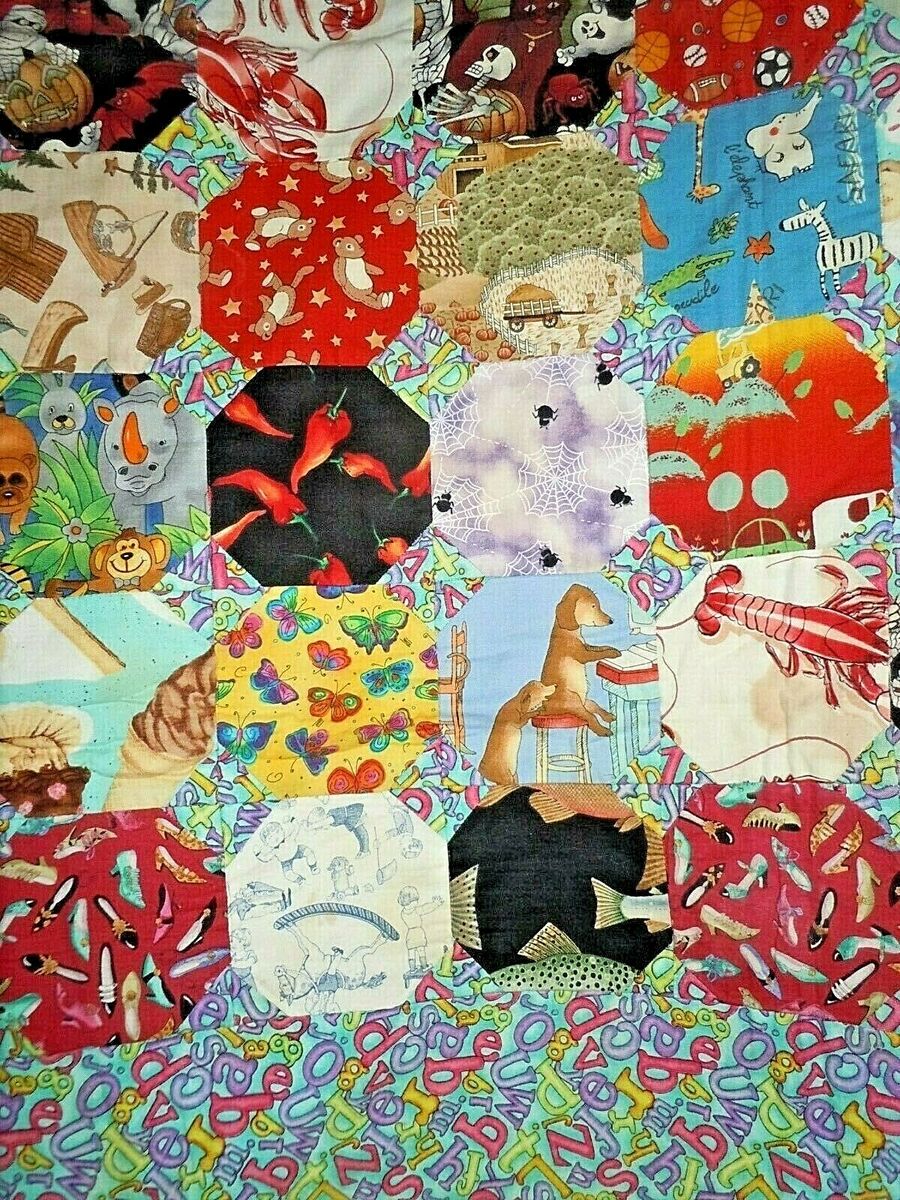The photograph captures a vibrant quilt composed of a blue fabric backing adorned with colorful alphabet letters in reds, yellows, purples, greens, and more. Each letter of the alphabet is represented, creating a lively and educational background. Attached to this backing, the quilt is further embellished with an array of 16 distinctive fabric squares arranged in four rows and four columns. 

Starting from the top left, the squares display a variety of whimsical and themed patterns. The first square features a tannish-gray fabric with outdoor gear motifs, including a boat with a fishing rod, a canoe, and a jacket. Adjacent to that is a red fabric filled with charming teddy bears. Other panels showcase a red chili peppers pattern on a black background, dogs working on typewriters, a bright red lobster, colorful butterflies, and sports equipment. Additional squares depict a playful car, a whimsical zebra, spooky ghosts, a rugged rhinoceros, a lively monkey, and a mummy dressed for Halloween.

Each section contributes its unique narrative, creating a rich tapestry that merges both aesthetic appeal and a touch of storytelling. This quilt is not just a cozy covering but a vivid patchwork of life’s diverse elements, making it a meticulously detailed and enchanting piece.